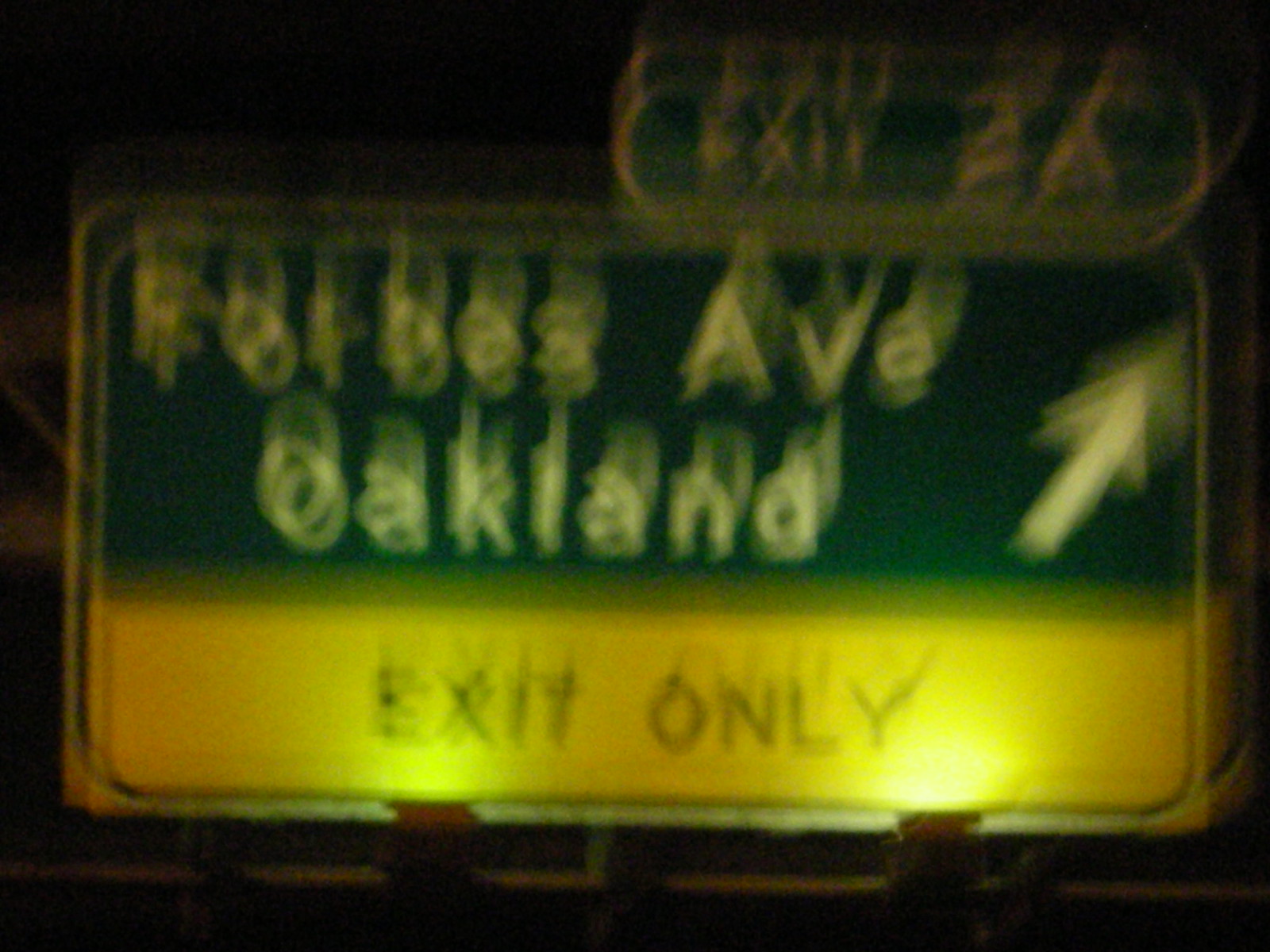This image, taken at night and somewhat blurry, features a standard rectangular highway exit sign. The sign consists of a green top section with white text that reads "Forbes Ave Oakland" and a large white arrow pointing diagonally to the right. The bottom portion of the sign is yellow with black text stating "exit only". Above the main sign, there's a smaller green sign with a white border, which appears to indicate "Exit 2A", although it is quite blurry. The sign is illuminated by two spotlights, enhancing visibility for nighttime drivers. The close-up nature of the photo, likely taken while driving, emphasizes the sign’s metallic structure and typical design found on highways across the United States.